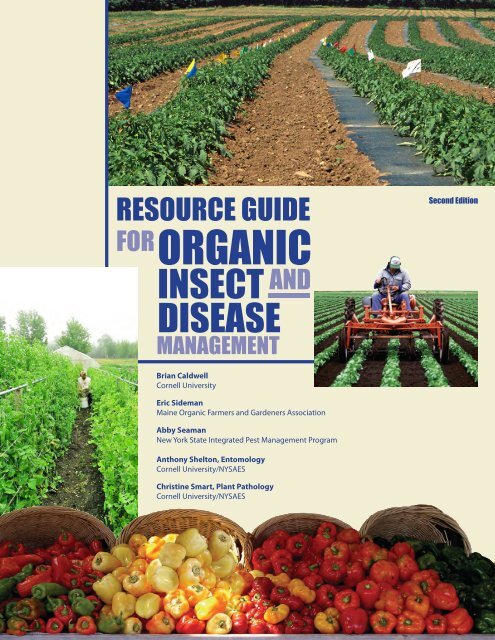The cover of the "Resource Guide for Organic Insect and Disease Management, Second Edition" features a vibrant, informative layout. At the top, a large photograph captures a field with alternating strips of green plants, brown dirt, and areas covered with black plastic. Scattered within the greenery, small flag markers stand out. Just beneath this, another image showcases a farm worker driving a red tractor through a lush, well-maintained field. On the left side, yet another image depicts a person wearing a cap and tending to an overgrown field, possibly near a greenhouse.

Dominating the center of the cover, in blue font, the title "Resource Guide for Organic Insect and Disease Management" is prominently displayed. Below the title, the authors are listed: Brian Caldwell from Cornell University, Eric Seidman from the Marine Organic Farmers and Gardeners Association, Abby Seaman from the New York State Integrated Pest Management Program, Anthony Shelton from the Entomology department at Cornell University and NYSAES, and Christine Smart from the Plant Pathology department at Cornell University and NYSAES.

At the bottom, a colorful arrangement of four tipped-over bushel baskets spills out a bounty of red, green, yellow, and orange peppers, emphasizing the organic focus of the guide. This visually appealing and detailed cover effectively communicates its purpose and invites readers into the world of organic farming and pest management.